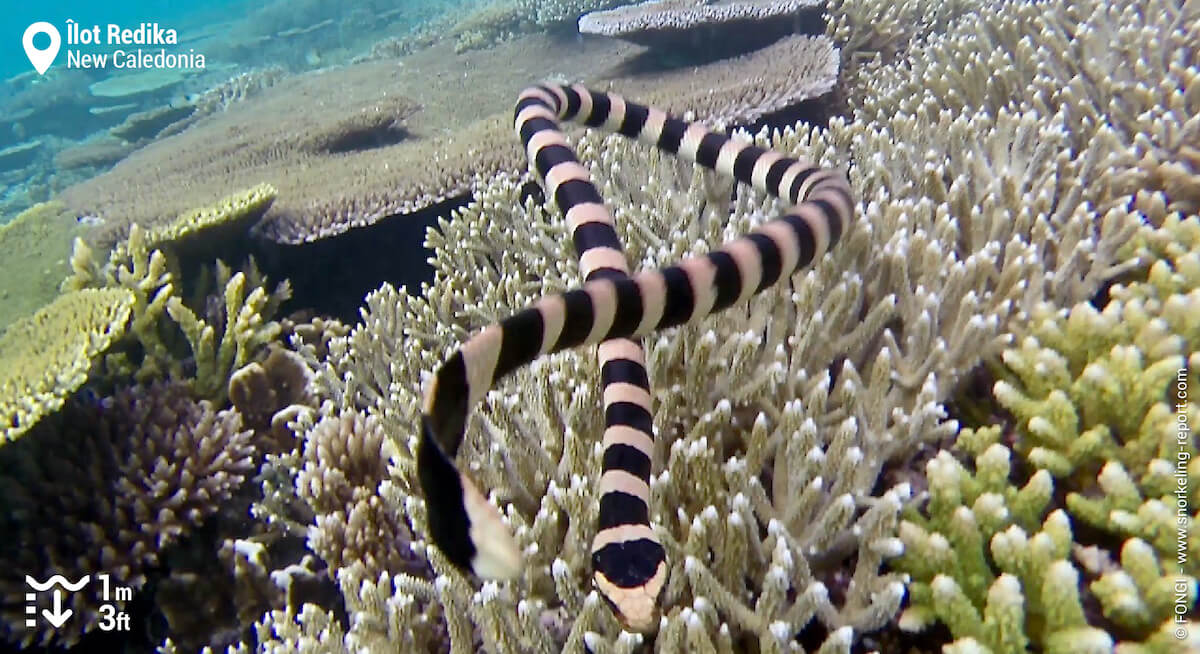This underwater photograph captures the vibrant ecosystem of a coral reef in New Caledonia. Dominating the center of the image is a striking cream and black-striped sea snake, its body curled into a figure-eight with its head facing the viewer and tail looping back near its head. The reef features a diverse array of corals, including flat saucer-like green coral with stem-like bases and branching corals that project in various directions, also green in color. A prominent bed of white, candlestick-like corals stretches diagonally from left to right, while a small patch of light green, branch-like coral with cream-colored tips nestles in the bottom right corner. In the upper left corner, the vivid blue aqua water provides a contrasting backdrop. Text in the top left corner reads "Ilot Redica, New Caledonia" in white letters, and the bottom left corner displays an icon with a downward arrow and the measurement "1M 3FT," indicating the water depth.